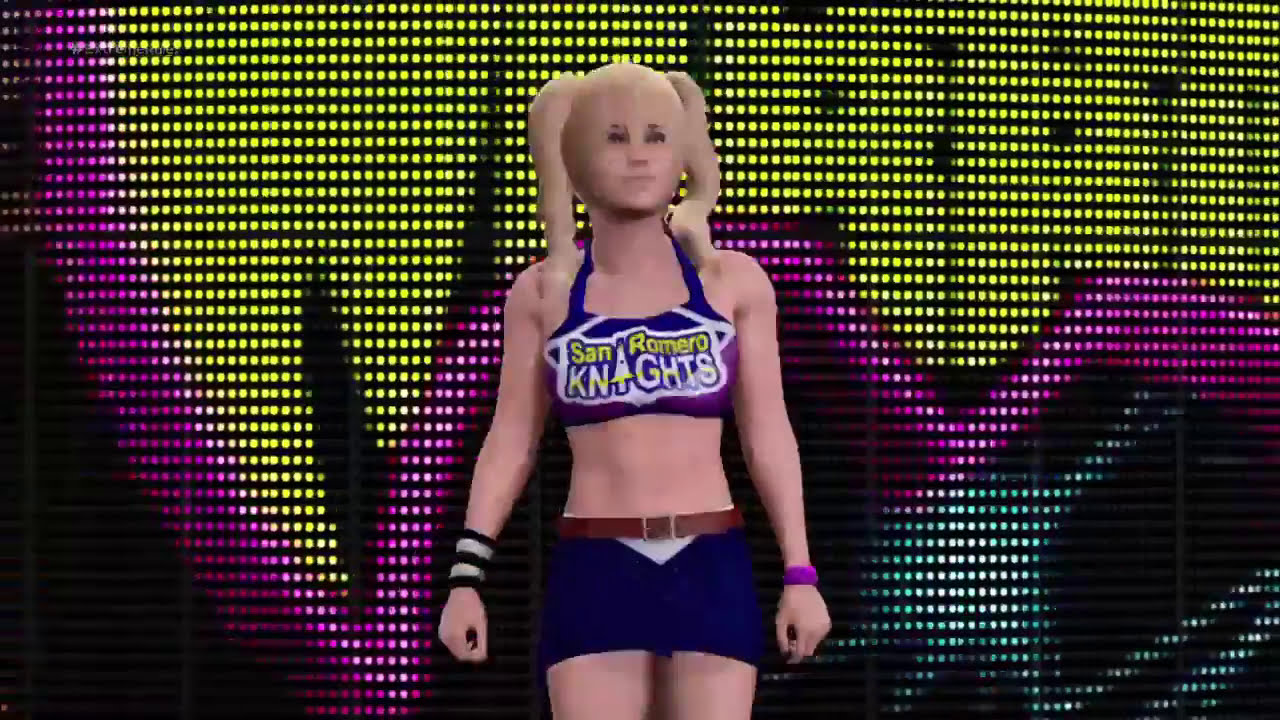This image is a detailed screenshot from a WWE-style video game, featuring a blonde female character positioned at the center. She has white skin and her hair is styled into pigtails that drape down to her shoulders. She is dressed in a blue and purple sporty half t-shirt that resembles a fitness bra, displaying the words "San Romero Knights". The text "San Romero" is yellow, and "Knights" is in white with a yellow stripe, including a distinctive sword-like design on the letter "i". She wears a blue mini skirt accompanied by a brown leather belt, and has bands on both her hands. Behind her, a massive LED screen forms the backdrop, adorned with a complex design featuring pink, yellow, and purple hues, possibly incorporating elements related to the Ultimate Warrior's logo. The LED screen's intricate pixel structure contributes to a dynamic entrance scene for the character in the game.